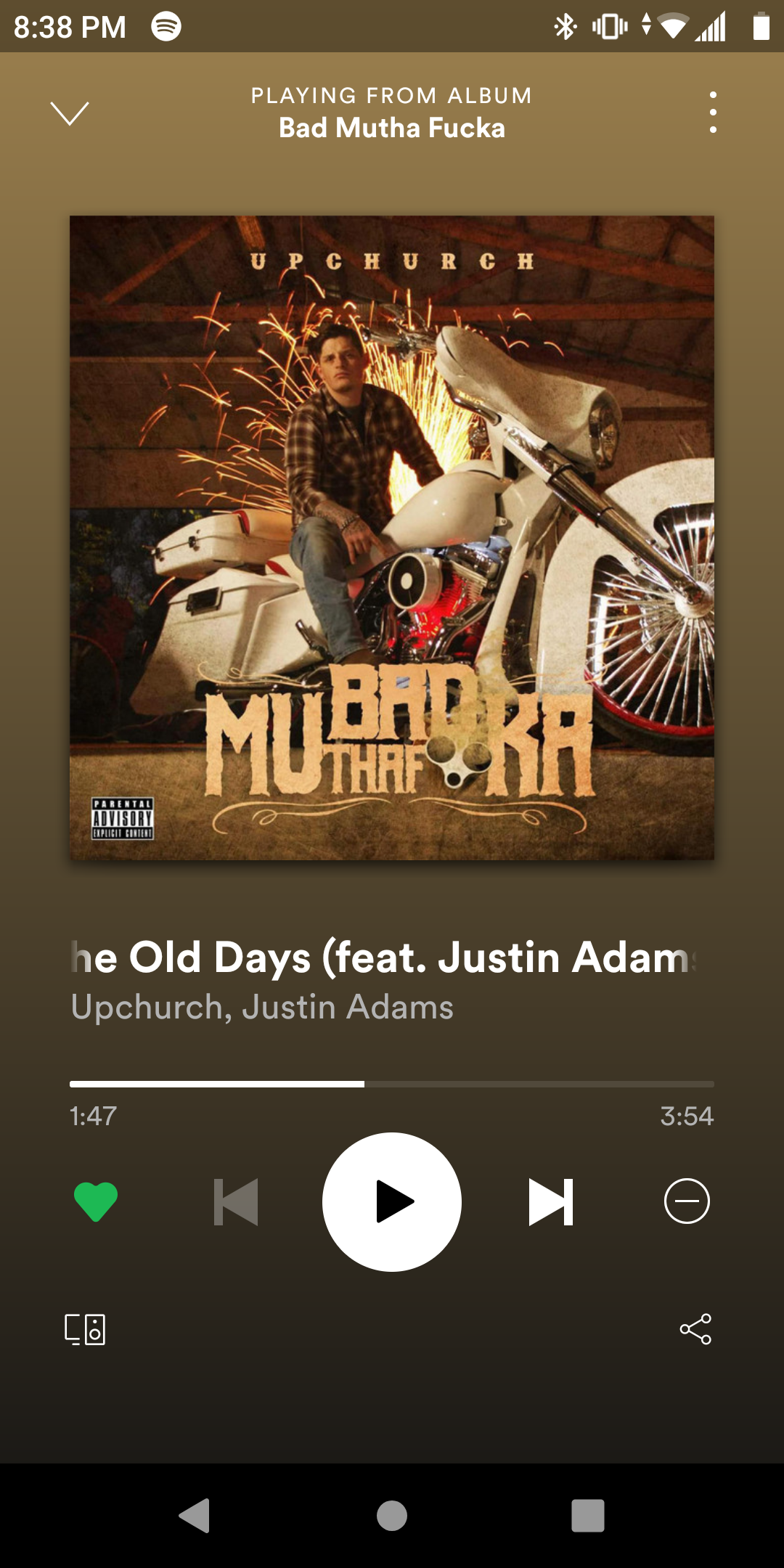The image depicts an Android phone display at 8:38 PM, showing the song "Bad Motherfucker" by Upchurch from a playlist, possibly on Spotify. The background of the phone screen features a striking ombre gradient, predominantly brown in color. The song is paused at 1:47 and marked with a heart icon, indicating it's a favored track. The album or song cover artwork showcased on the phone screen captures a rugged scene: a man clad in jeans and a flannel shirt sits atop an elaborately styled white motorcycle, complete with silver spokes and a large trailer-like attachment at the rear. The setting appears to be inside a barn, with dramatic welding sparks illuminating the background, adding a touch of dynamic intensity to the image.